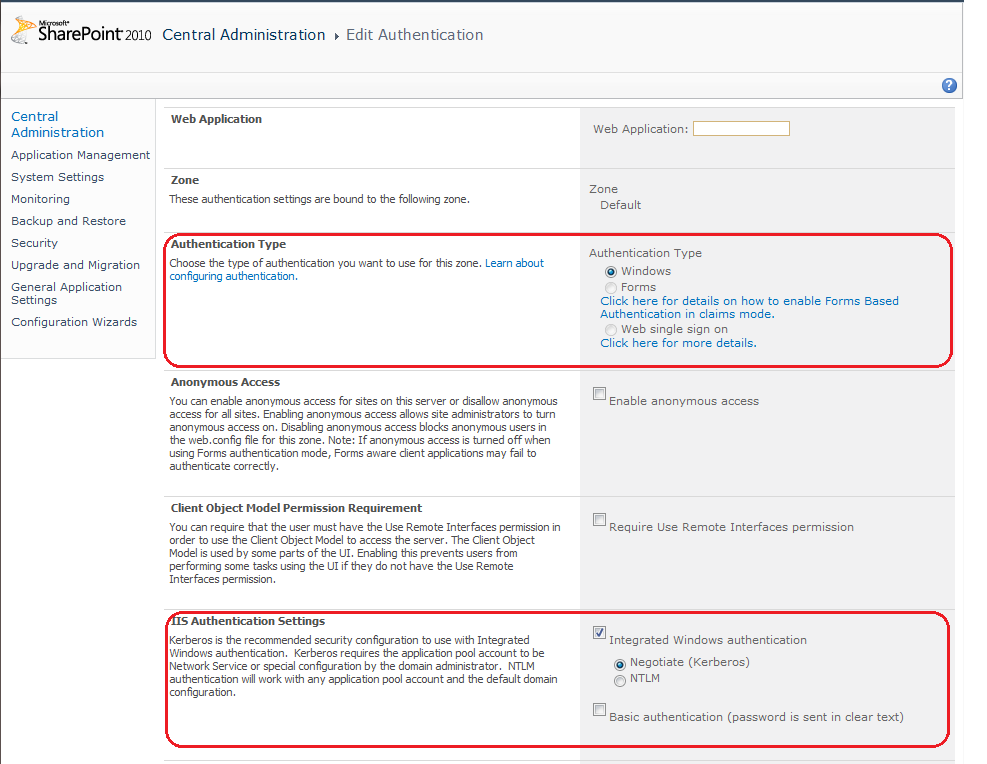This screenshot showcases the Microsoft SharePoint 2010 Central Administration interface. The top of the screen features a light gray background with a navigation path text that reads "Microsoft SharePoint 2010, Central Administration, Edit, Authentication" from the left edge. 

The interface is divided into vertical sections with white and gray backgrounds. On the far left, a side panel lists options for various administrative categories: "Central Administration," "Application Management," "System Settings," "Monitoring," "Backup and Restore," "Security," "Upgrade and Migration," "General Application Settings," and "Configuration Wizards."

To the right, there is a section titled "Select the Web Application." Under the heading "Zone," it states, "These authentication settings are bound to the following zone," specifying that the zone is "Default." For "Authentication Type," there is a prompt to choose the type of authentication for this zone, with an option to learn more about configuring authentication.

The current authentication type is set to "Windows," with additional options available for "Forms" and "Web Single Sign-On." Below these settings, there are further options for "Anonymous Access," "Client Object Model Permission Requirement," and "IIS Authentication Settings."